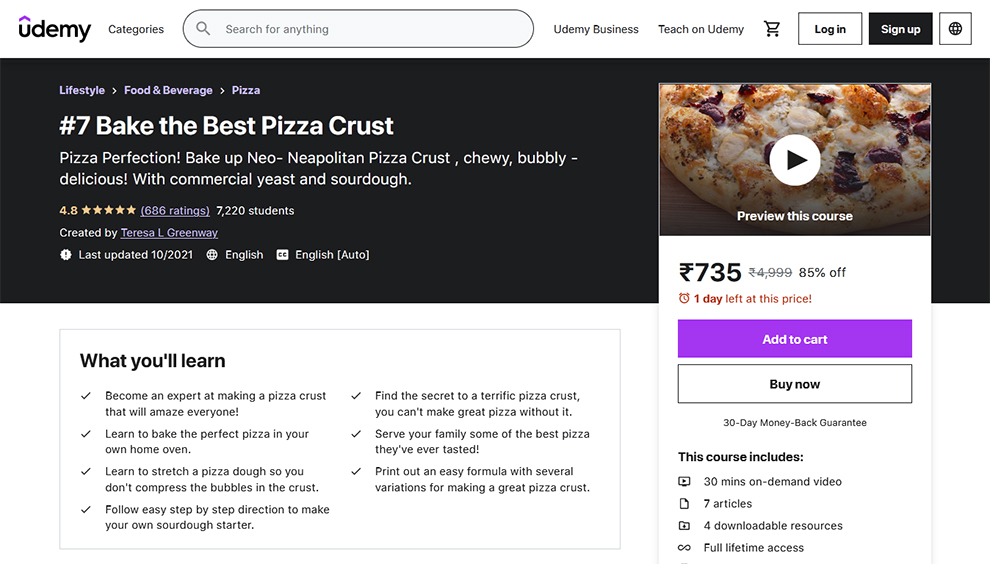This image is a detailed screenshot from the Udemy Learning Academy's webpage showcasing a specific course titled "Bake the Best Pizza Crust." 

At the top of the screenshot, there are several navigational features including:
- Categories
- A search field with a capsule-shaped outline
- Udemy Business
- Teach on Udemy
- Shopping Cart
- Login
- Sign Up
- A gear icon for settings

Below this header, a large black banner displays "Lifestyle, Food and Beverages, Pizza." Further down, the course details are prominently featured with the title "Bake the Best Pizza Crust" alongside a descriptive tagline: "Pizza Perfection: Bake a Neapolitan Pizza Crust, Chewy, Bubbly, Delicious, with Commercial Yeast and Sourdough." The course boasts a 4.8-star rating based on 686 reviews and is popular with 7,320 students enrolled. Created by Teresa Greenway, the course was last updated on October 20, 2021, and is available in English, with English auto-generated subtitles.

To the right, there's an image featuring a pizza with a play button overlay, inviting users to preview the course. The course is priced at 735 (currency unspecified), currently at an 85% discount, with one day left at this promotional price. Options to "Add to Cart" (highlighted in purple) or "Buy Now" are also available.

Below this, there is a summary of what participants will learn, including:
- Becoming an expert at making pizza crust
- Learning to bake the perfect crust

The course includes:
- 30 minutes of on-demand video
- 7 articles
- 4 downloadable resources
- Full lifetime access

This detailed and visually organized layout provides prospective students with all the essential information they need to make an informed decision.